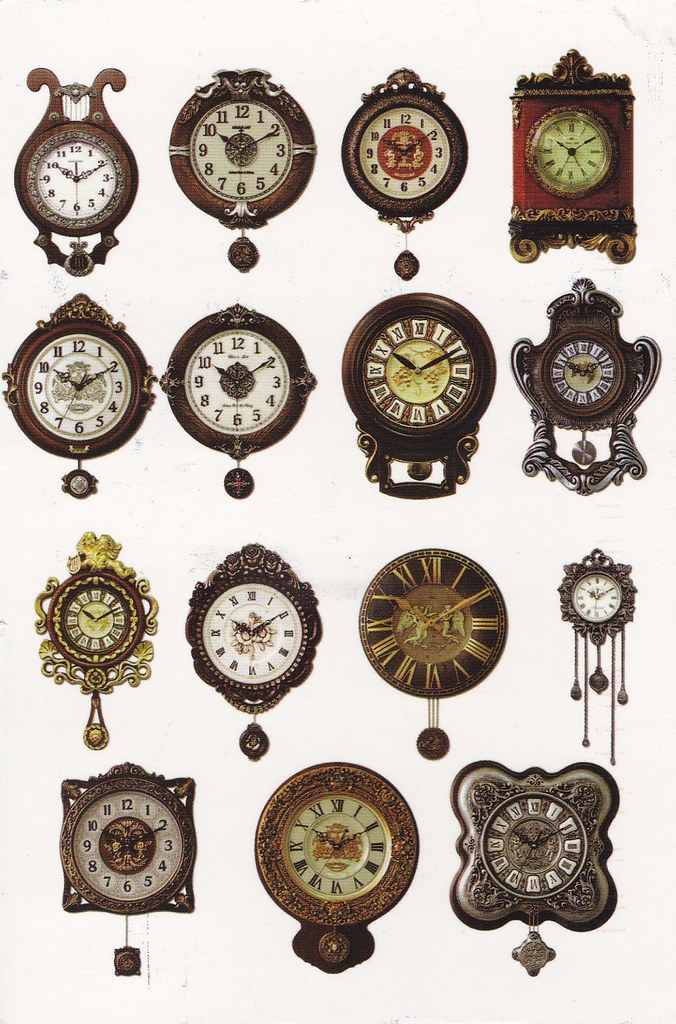This photograph showcases an exquisite collection of 15 antique clocks meticulously arranged in a grid format, with four rows of four clocks each and an additional three clocks at the bottom. These clocks, ranging from Baroque to 19th-century styles, boast incredibly ornate frames with elaborate scrollwork, flowery designs, and intricate flourishes that elevate their antique allure. The majority feature round faces, although there is at least one rectangular clock encased in wood, adding a unique dimension to the collection. The faces of most clocks display Roman numerals, while a significant number utilize standard Arabic numerals. Predominantly crafted in shades of gold, brown, bronze, and silver, each clock exudes a sense of opulence. All but one of the clocks dangle long pendulums, further enhancing their old-fashioned charm. Despite their age, the faces of these timepieces remain light-colored for easy readability, emphasizing their functional beauty.